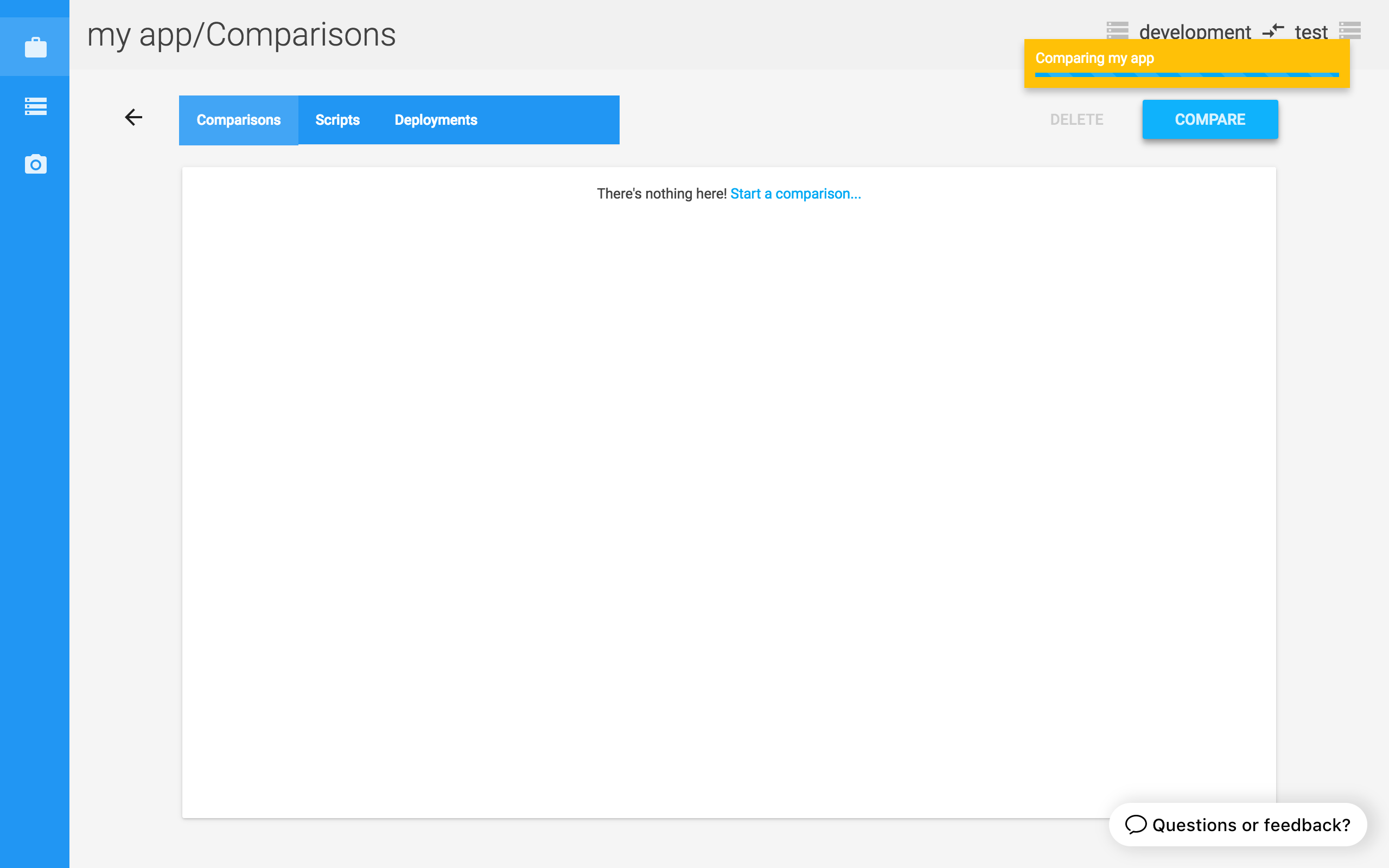A detailed screen capture from the "Comparisons" section of the user's app, labeled "Comparisons" with a captial "C". At the top right, there are menu options for "Development" and "Test." Below these menus, a yellow status bar with a nearly complete blue progress line (approximately 99%) stretches across the screen, displaying the message "Comparing my app." 

On the top left, below the app name, there are three selectable buttons: "Comparisons," "Scripts," and "Deployments," with "Comparisons" currently highlighted. Beneath these buttons, a large white area dominates the screen, featuring a prompt at the top that reads, "There's nothing here. Start a comparison."

On the far right bottom corner of the screen, a dialog box is available for submitting questions or feedback. Running vertically along the left side of the screen is a blue banner containing icons for "Folders," "Menu Choices," and "Camera," providing quick navigation options.